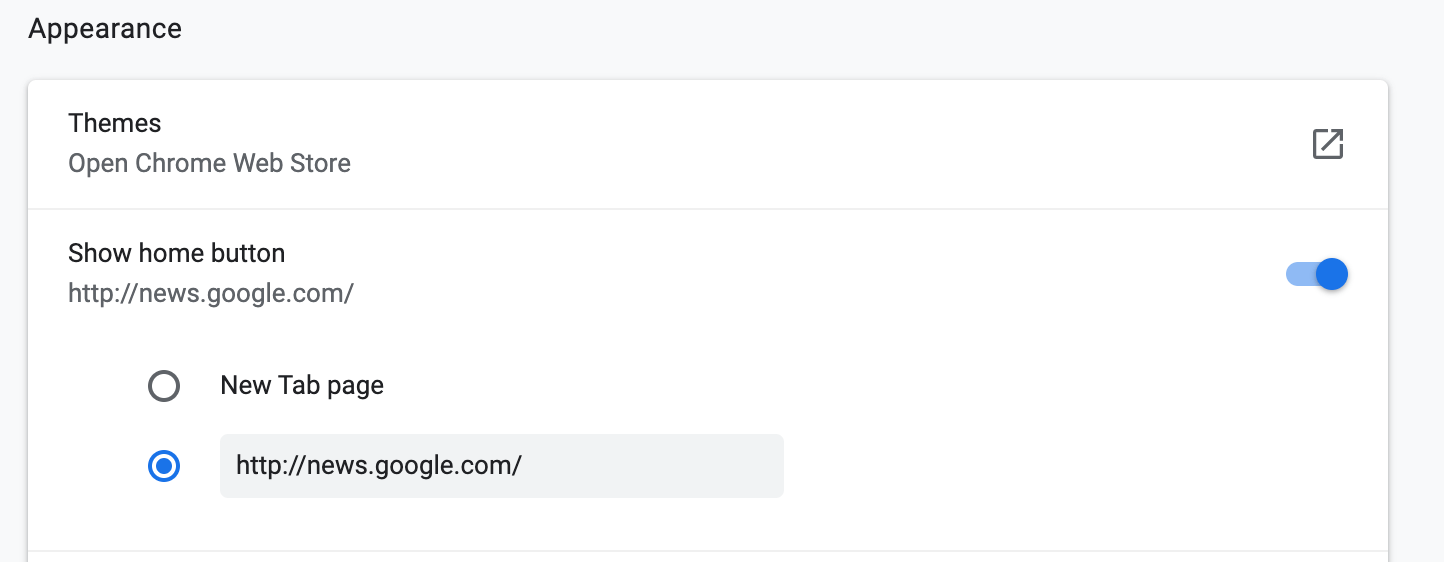A screenshot detail captures a section of a browser's appearance settings interface. At the top left, the term "Appearance" is displayed in dark grey font, set against a dark, light grey background. Below this, against a predominantly white background, is the header "Themes," followed by a link labeled "Open Chrome Web Store." To the right of the phrases 'Themes' and 'Open Chrome Web Store,' there's a square icon featuring a diagonal arrow pointing to the top right, indicating a shortcut.

Underneath these elements, a heading labeled "Show Home Button" is present, with a toggle button beside it indicating it is turned on. This activated state is shown by a blue circle positioned to the right, leaving a trail of light blue to the left. 

Beneath the "Show Home Button" heading, there's a URL displayed: "http://news.google.com/". Further down, there are two radio buttons. The first option is "New Tab Page," and the second option is another instance of "http://news.google.com/". The latter is selected, indicated by a small blue circle within the radio button. This text is set inside a light grey rectangle.